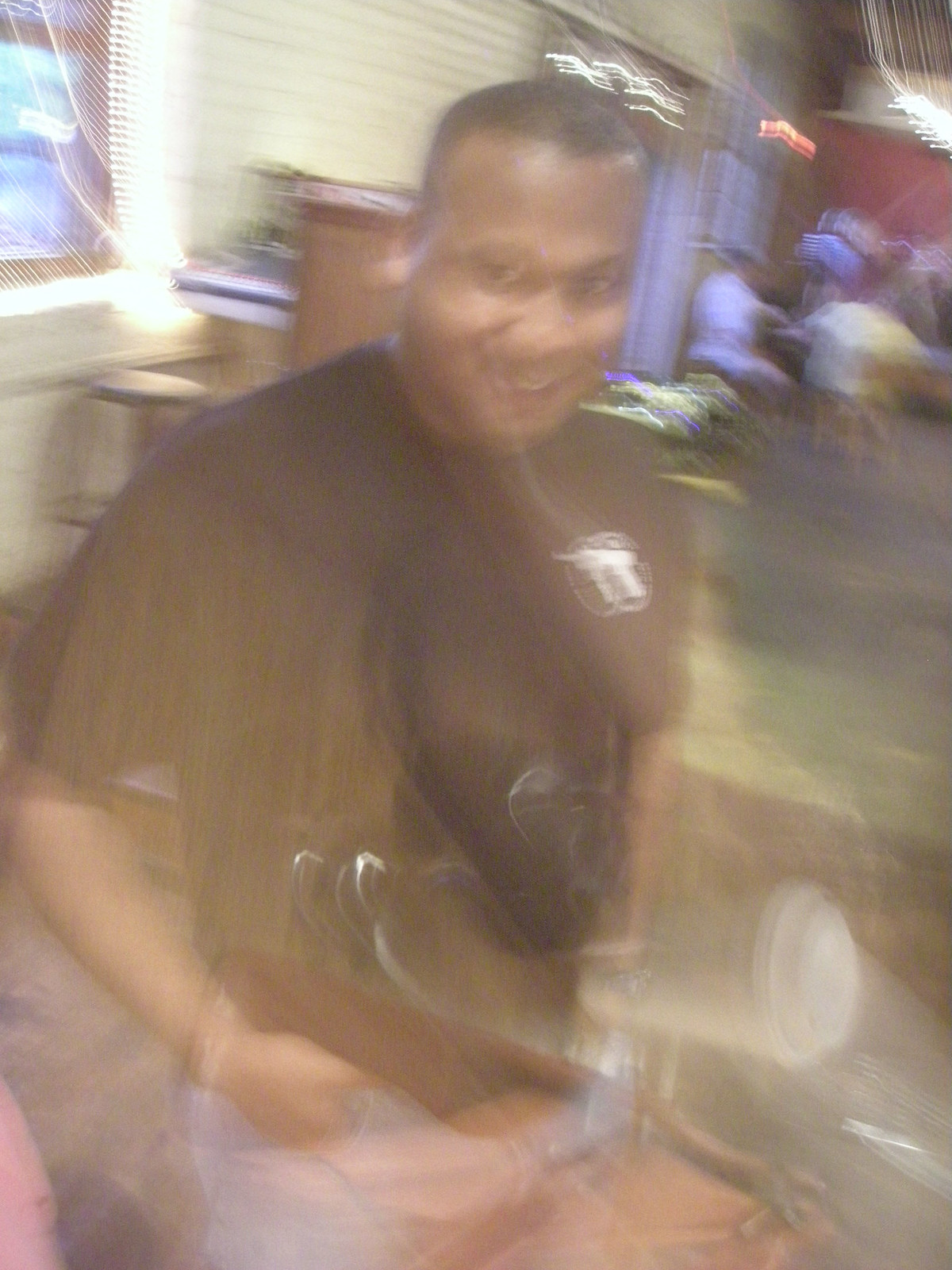This photograph is heavily blurred, making it difficult to discern distinct elements clearly. However, it appears to depict a black man smiling at the photographer while lying on his side. He is dressed in a black t-shirt adorned with a white logo on the left breast and is wearing blue jeans. A watch is visible on his right wrist. There is an unclear artifact around his neck that might be a camera strap, though this is uncertain due to the overall poor quality of the image.

There is also a takeaway coffee cup with a lid emerging from his stomach area, strongly suggesting that the photo may be an overlay of two different images. This theory is supported by another noticeable artifact that resembles an additional photographic element.

In the background, there is a cream-colored building with a window, and in the top right corner, several people are seated at tables, adding to the scene. Despite the heavy blurring, these details combine to form a complex, though confused, visual narrative.